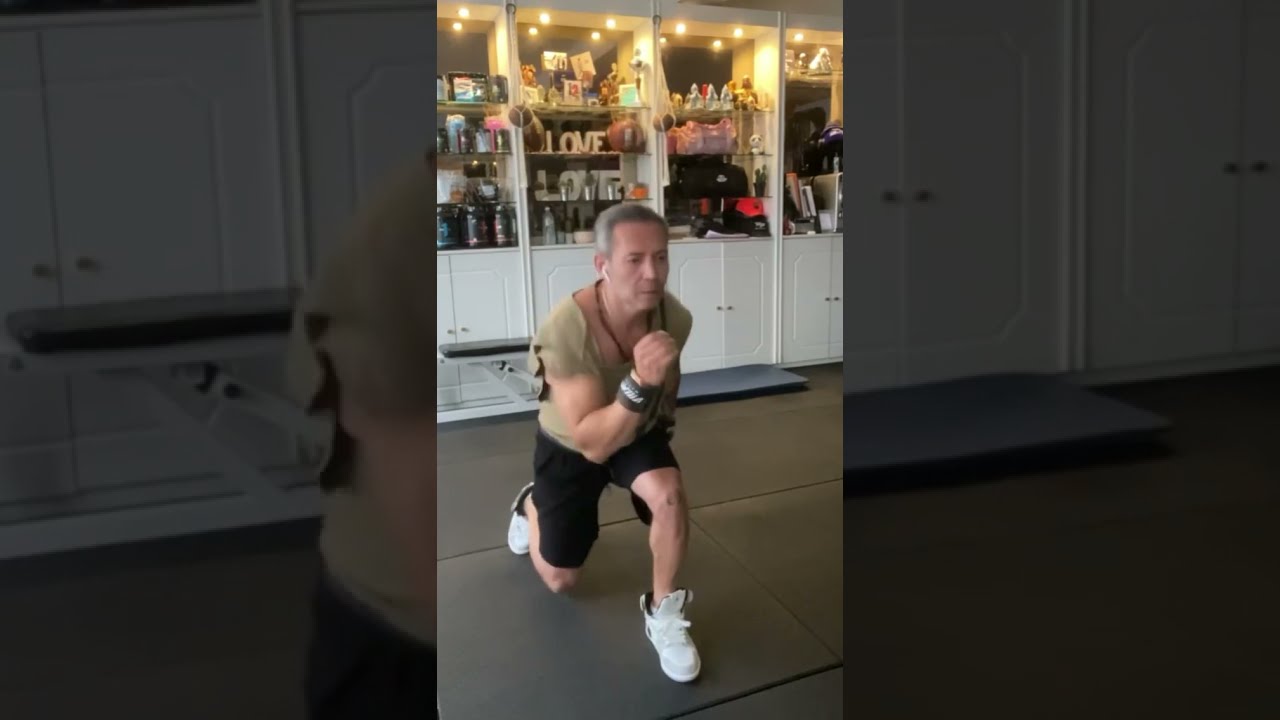In the central vertical rectangle of this color photograph, inset against a darker, enlarged landscape orientation of the same image, a fair-skinned, muscular man with short gray hair is captured in the middle of an active workout routine indoors. He is lunging forward, with his left leg bent at the knee and his right leg stretched back, his right arm forward and left arm back, poised in a strong exercise stance. The man is wearing a loose-fitted, greenish shirt with cut-out sleeves and collar, black athletic shorts, and white tennis shoes. Around his neck, there's a red band, and white earbuds are in his ears. The floor beneath him is covered with black rubber mats or yoga mats. Behind him, white cabinetry occupies the lower part of the wall, while open shelves with various knickknacks, statues, and picture frames line the upper section, illuminated by small overhead lights. The word "LOVE" is spelled out in block letters on two of the shelves. The photograph's app screenshot format includes faded and darkened repetitions of the image on the left and right sides, providing a close-up view of the man's back and the cabinetry.